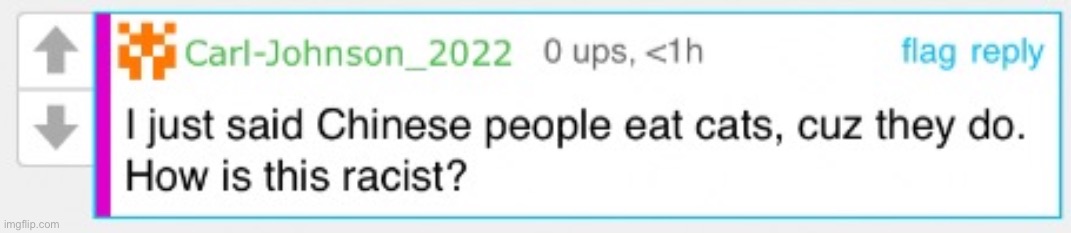This image is a screenshot of an online message. On the left side, there's a gray sidebar with two squares, one above the other. The upper square features an upward arrow, while the bottom square has a downward arrow, both in medium gray.

Next to the sidebar, there is a banner in a medium purple hue with hints of pink or red, bordered by a thin blue line. The banner includes an orange graphic resembling a digital robot. Adjacent to the graphic, green text reads "Carlts-Johnson_2022." Below this, gray text states "0 UPS, 1 hour." Over to the right, "flag reply" appears in blue text.

Beneath this banner is a black-printed message that reads: "I just said, 'Chinese people eat cats, cuz they do. How is this racist?'" Note that "Chinese" begins with a capital C, "cuz" is spelled C-U-Z, and "How" starts with a capital H.